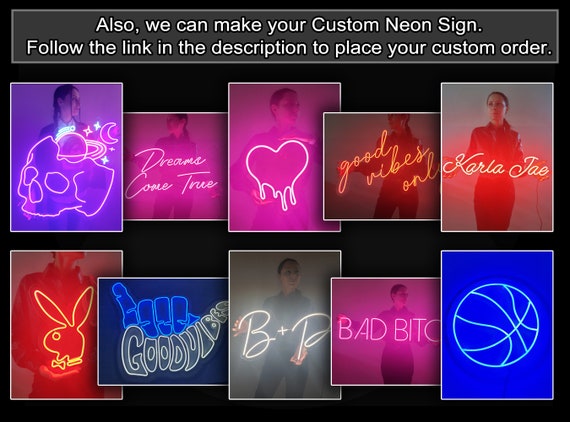This horizontal, rectangular advertisement for a neon sign company features ten different neon signs in various colors, all inset against a black background. At the top, white text reads, "Also, we can make your custom neon sign. Follow the link in the description to place your custom order." The signs are displayed in two rows. 

In the top row, from left to right, there is a pink neon sign depicting a skull with a ringed planet emerging from the top, followed by pink text that reads "Dreams come true." Next is a pink heart melting at the bottom, orange text reading "Good vibes all," and an orange sign with the name "Carla J."

In the bottom row, the leftmost sign is an orange Playboy Bunny logo, followed by a blue hang ten sign showing a fist, with the white text "Good vibes" beneath it. Next is white text reading "B + P," pink text of "Bad Bitch," and a blue basketball.